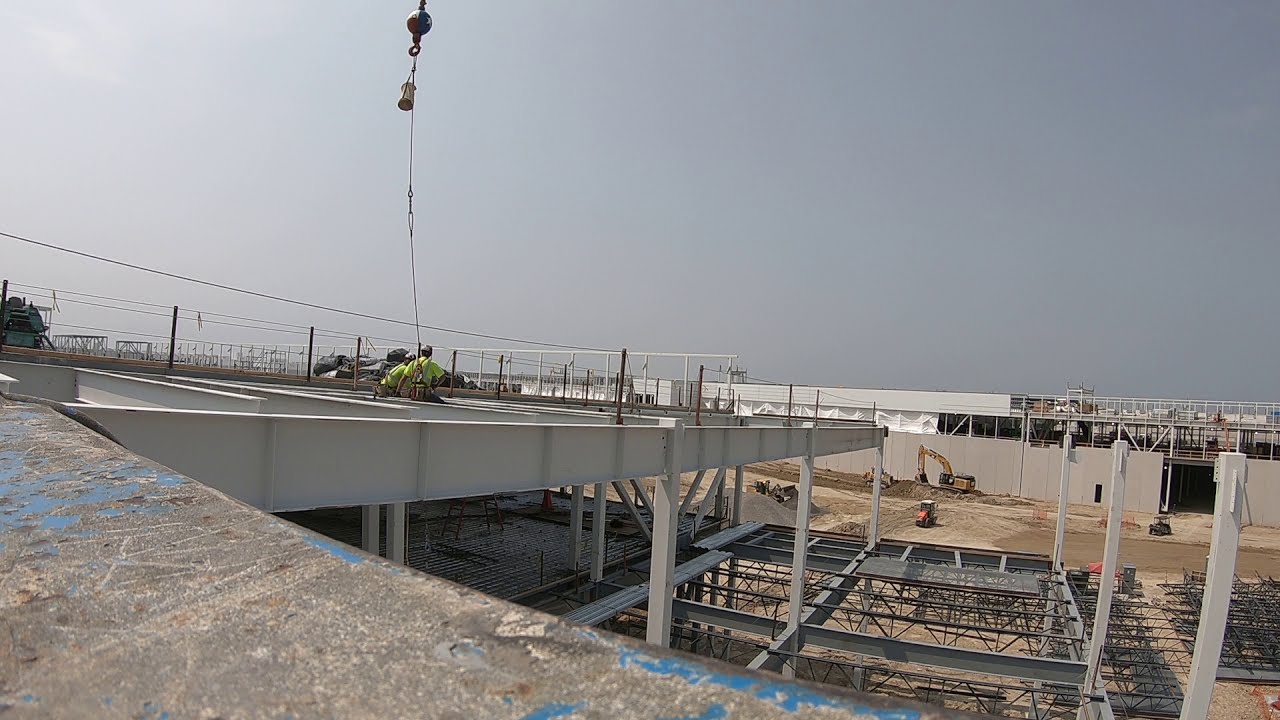The image depicts an expansive outdoor construction site set under a deep gray sky, potentially signaling an approaching storm. The setting includes a wide-open industrial area with a lot of concrete, indicative of ongoing large-scale construction or industrial work. In the foreground, on top of a concrete pillar or a partially constructed building with visible metal frameworks and scaffolding, two construction workers can be seen wearing bright yellow safety shirts and hard hats. They are standing near a large crane, which is hanging from the top of the frame, holding a bucket with a strap. Surrounding the workers are a variety of construction elements, including beams, steel structures, and a significant amount of dirt, contributing to the overall industrial ambiance. There are also construction vehicles, including a large one and smaller golf cart-like vehicles, maneuvering the dirt. The site is enclosed by fences, gates, and orange safety cones, emphasizing the ongoing construction work and the safety precautions in place.